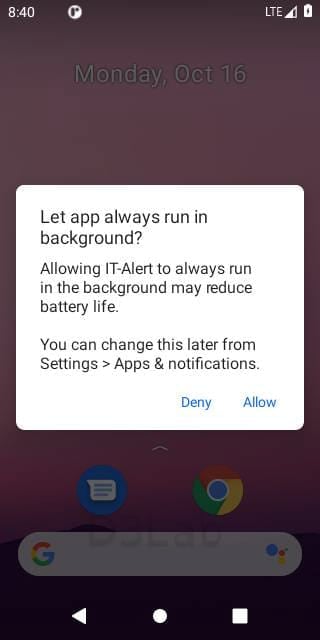**Detailed Caption:**

This image is a mobile screenshot showcasing a screen with a dark magenta gradient background at the top, transitioning to black towards the bottom. At the top of the screen, in translucent text, the date "Monday, October 16th" is displayed. Adjacent to the left side, there is additional information including the time "8:40 AM," and network status "LTE" accompanied by two small icons on the upper right corner.

The center upper portion features a prominent, large white text box with the message: "Let app always run in background. Allowing IT alert to always run in the background may reduce battery life. You can change this later from settings > apps and notifications." This message is accompanied by two interactive options: a "Deny" button and a "Allow" blue-text link located in the lower right corner of the text box.

Towards the bottom of the screen, faintly visible in translucent overlay, are three primary elements. First is a messaging icon, followed by a Google Chrome icon, and a Google search box that features the Google "G" logo on the left and an additional colored icon on the right. Superimposed on the upper portion of the Google search box is some light gray, oddly stylized translucent text.

Finally, at the very bottom of the screen are three standard navigational icons: a white triangle pointing left, a white circle, and a white square, offering navigation commands for the user.